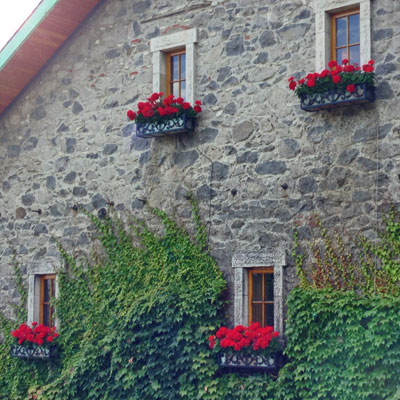This image captures the side of a two-story stone house, composed of variously sized and textured stones in shades of light gray, dark gray, and tan. The sturdy construction is accented by the reddish-brown underside of the roof, which slants down from the top left corner. The house features four inset windows with wooden brown frames and decorative white trim. Each window is adorned with a window box filled with flourishing red flowers, possibly marigolds. The window boxes themselves are decorative, featuring hints of blue. Below the two lower windows, lush green ivy in two shades climbs the wall. The ivy on the left appears darker, while the right side is lighter, with some brownish hues mixed in as it ascends toward the second floor. The image, square in shape and taken outdoors during the daytime, shows a plain white sky in the upper left corner, providing a simple backdrop to the detailed features of the house.